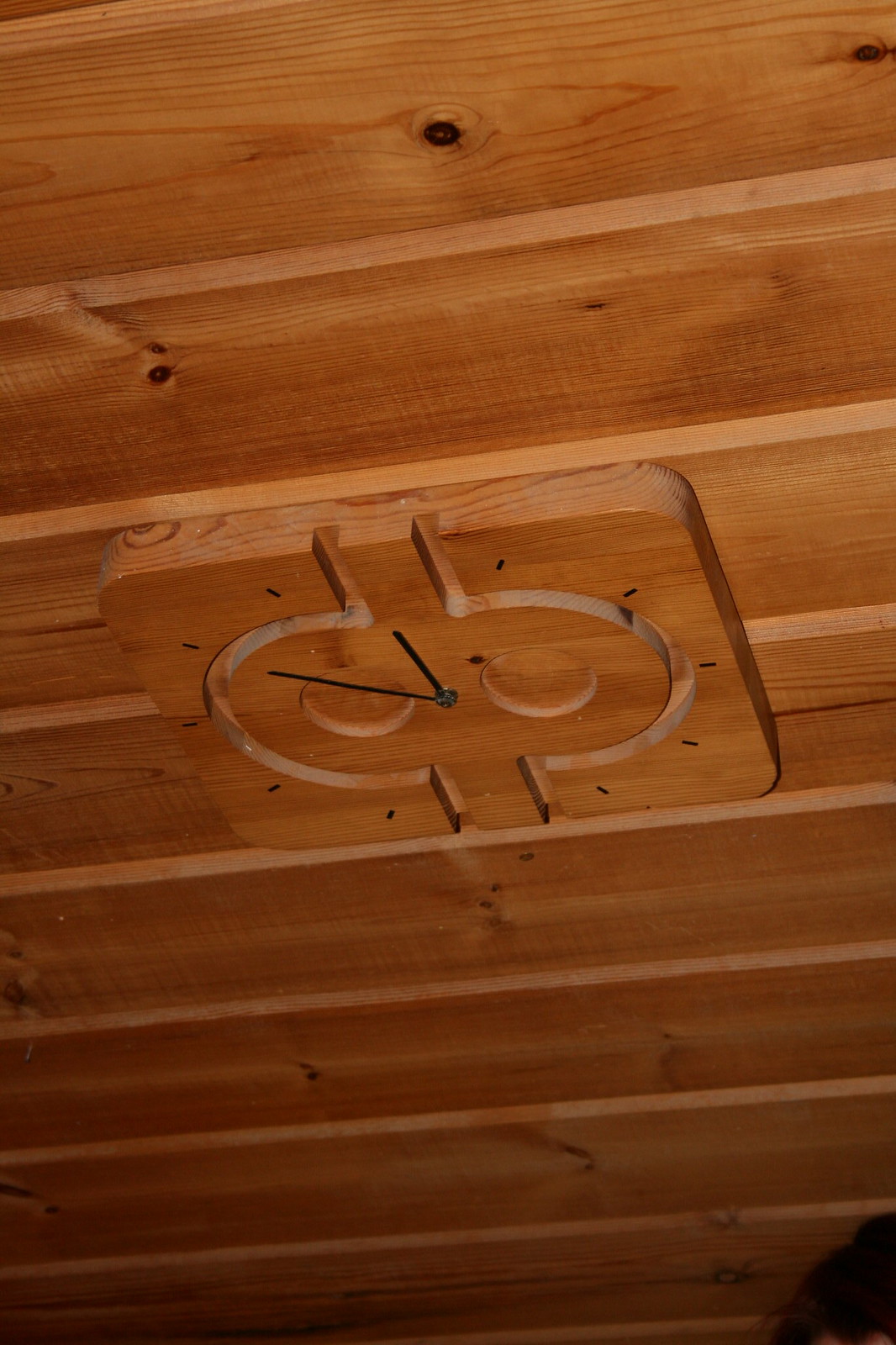The image depicts a unique and intriguing scene set against a wooden backdrop. Dominating the center of the photograph is a wooden block that seamlessly blends into the wooden surface with its matching texture and color. Embedded within this block is a clock face, meticulously designed with a semicircular array of time indicators. The clock face features two hands—one for the hour and one for the minute—both poised over the gradient markings that elegantly trace the semicircle's curve. The wooden background itself consists of several planks aligned with visible gaps between them, adding a rhythmic pattern to the composition. The angle from which the photo is taken lends a slightly disorienting yet captivating perspective, creating a visual puzzle as to the orientation of the elements on display.